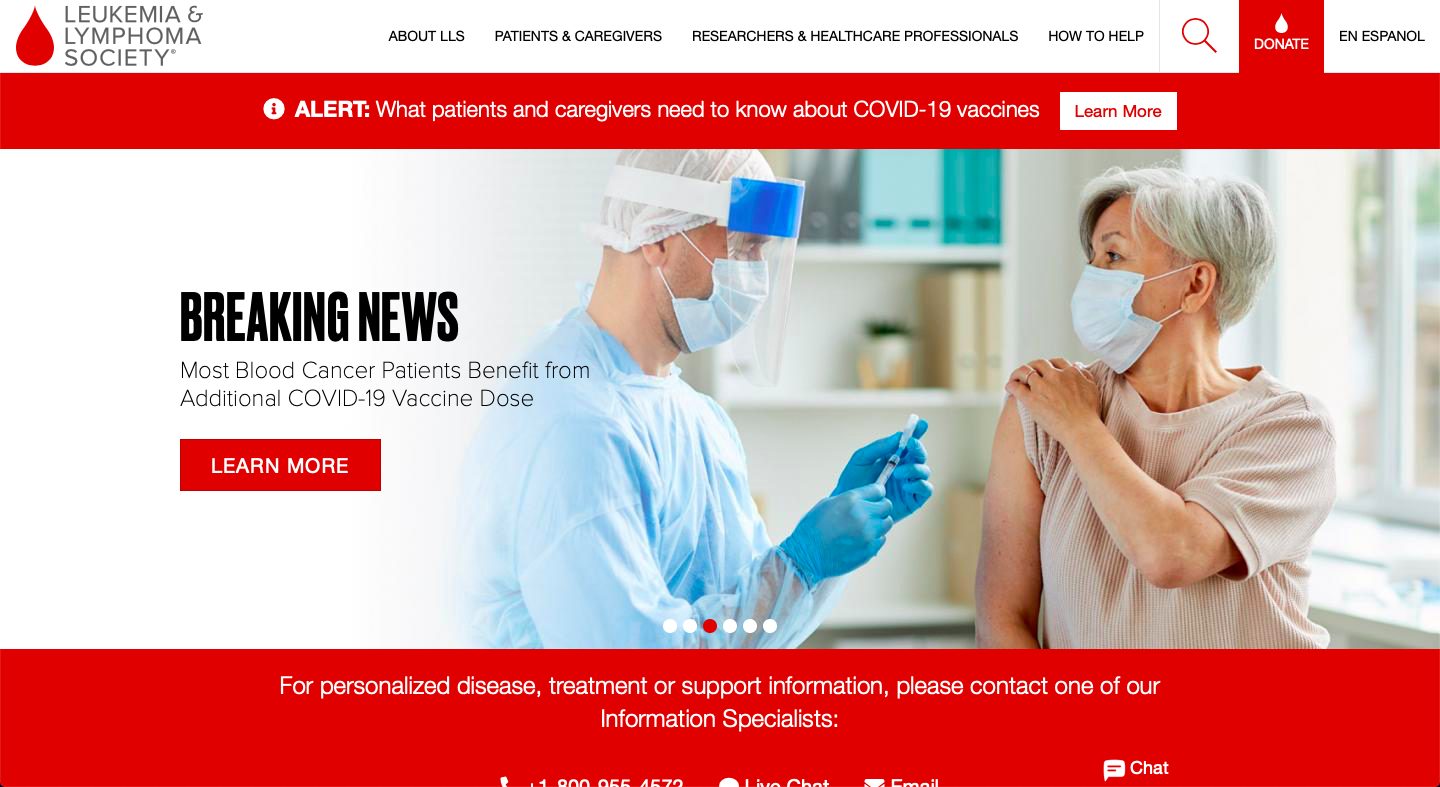**Descriptive Caption:**

This is a detailed screenshot of the Leukemia and Lymphoma Society (LLS) website. The logo on the left-hand side features the organization's name arranged in three lines: "Leukemia and" on the first line, "Lymphoma" on the second line, and "Society" on the third. Adjacent to the text is a blood droplet icon.

The website's top navigation bar includes headings in all caps and black font: "ABOUT LLS," "PATIENTS AND CAREGIVERS," "RESEARCHERS AND HEALTHCARE PROFESSIONALS," and "HOW TO HELP." There is also a white search bar with a red magnifying glass icon and a red "DONATE" button featuring a blood droplet symbol. On the far right side, there is a link labeled "EN ESPAÑOL" in black caps.

Below the navigation bar, a prominent red banner spans the width of the page. On the left side of the banner is a small white circle containing a lowercase "i." To its right, bold white capital letters spell out "ALERT," followed by white text reading, "What patients and caregivers need to know about COVID-19 vaccines." A "LEARN MORE" link is displayed in red text inside a white rectangle.

The central portion of the screenshot showcases an image of an elderly woman with short white hair, wearing a COVID-19 mask. She is lifting her sleeve as a healthcare professional, who is equipped with a mask and face shield, appears to be administering a vaccine. Accompanying the image is breaking news text stating that "Most blood cancer patients benefit from additional COVID-19 vaccine dose." A red "LEARN MORE" button provides further information.

At the bottom of the screenshot, a message encourages individuals seeking personalized disease treatment or support information to contact one of their information specialists.